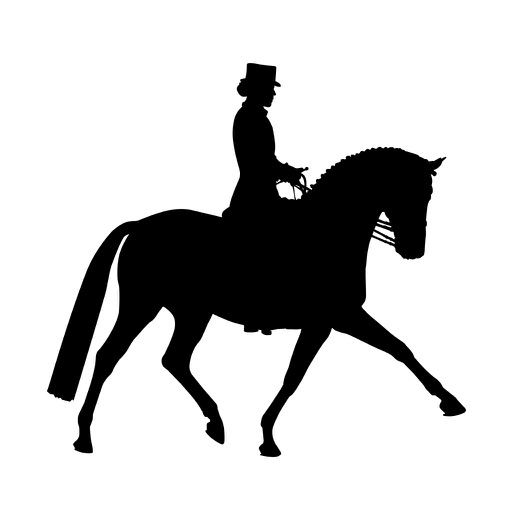The image features a solid black silhouette of a woman riding a horse, both seen in profile, facing to the right, against a white background. The woman appears to be elegantly dressed, wearing a top hat and formal attire, with her hair neatly styled in a bun. She is holding the reins with both hands positioned in front of her. The horse's mane is intricately braided, forming small, distinct bubbles along its back, and its long, well-maintained tail nearly reaches its legs. The horse appears to be in motion, lifting its front hoof as if trotting. The overall style suggests a refined and polished appearance for both the rider and the horse.